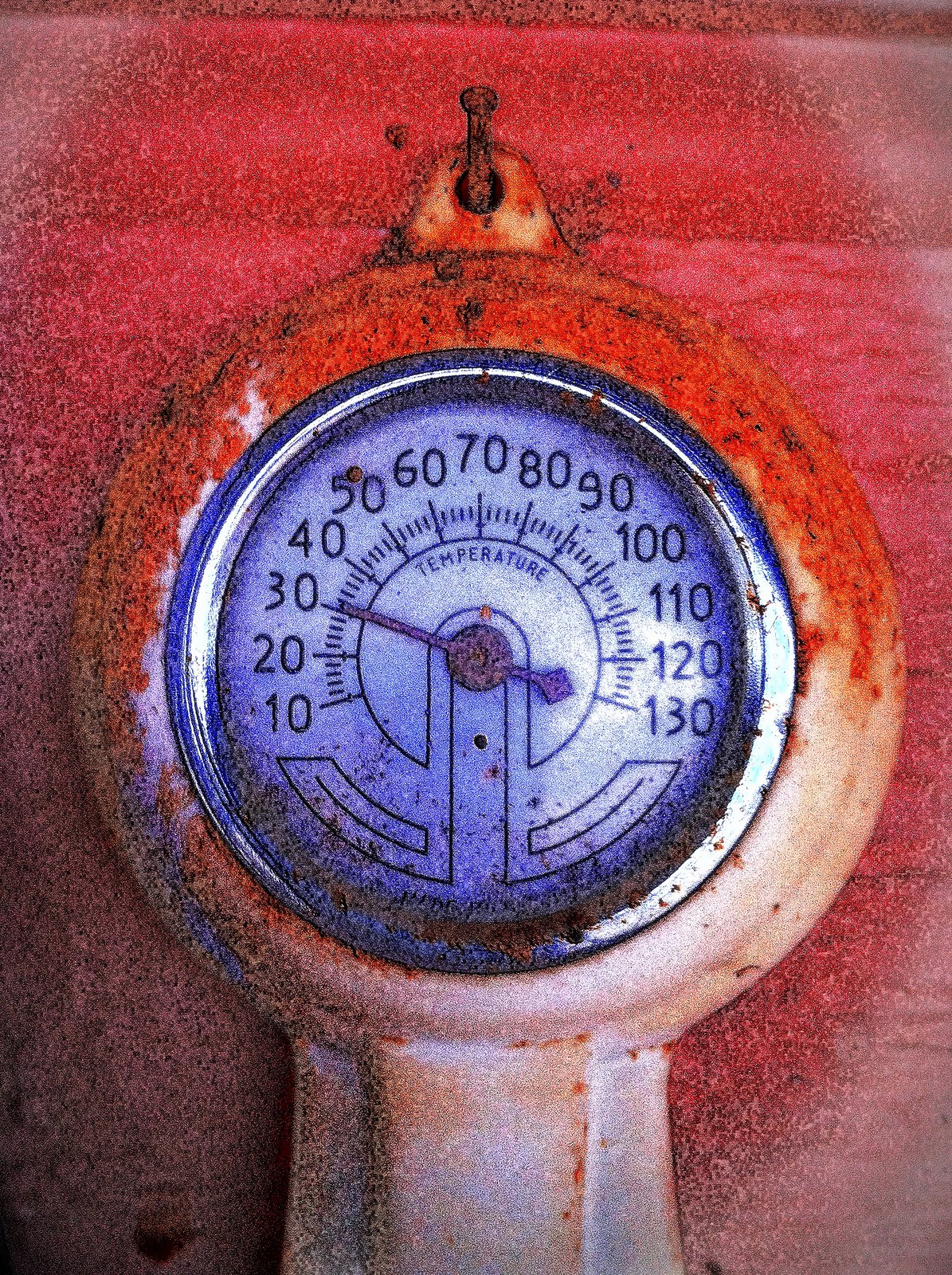Detailed Caption:

The image showcases a close-up of an old, weathered thermostat. The top portion of the thermostat appears rusted with a reddish hue, suggesting either significant oxidation or a red filter applied over the image. A purposeful hole at the top of the thermostat allows it to be mounted, currently hanging from a bent nail with its circular head visible.

The main body of the thermostat is distinctly circular. The upper section retains the rusted red appearance, while the lower half transitions to a silver tone marred with sporadic rust spots. The central section features a silver circular face displaying a series of numbers in black, ranging from 10 to 130 in increments of 10.

A prominent red pointer is fixed on the face, indicating a temperature reading of approximately 32 degrees. Above this pointer, in bold capital letters, the word "TEMPERATURE" is clearly printed. The background of the image appears predominantly red, with gradually lighter red gradients emerging at the upper left, upper right, and bottom right corners, implying either a red surface or the influence of a red filter.

Below the circular part of the thermostat, the structure extends downward, starting to form a rectangular base. This section is also silver with scattered rust spots, but its full extent is not visible as it is cropped out of the image frame.